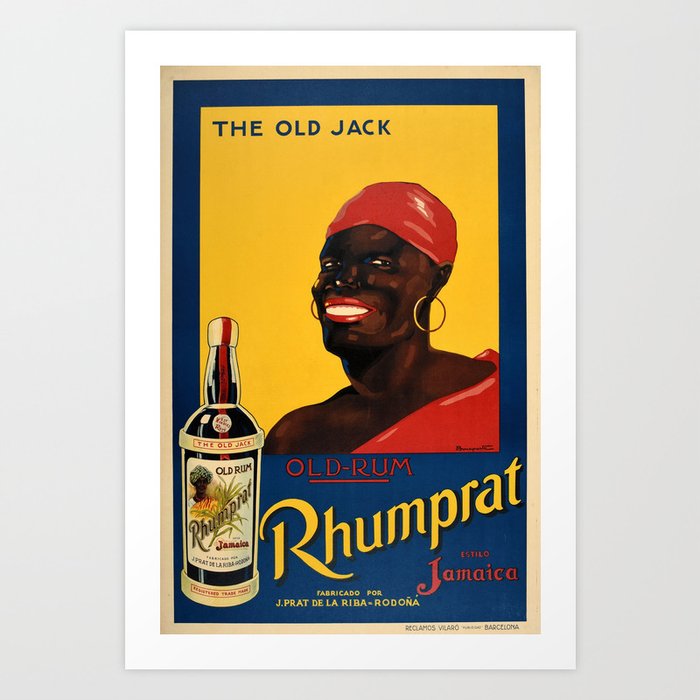The image is a vintage-style advertisement poster for a type of rum, mounted on a gray wall with a white mat border. This border is followed by a thin cream-colored mat, adding to its antiquated look. The poster itself is vertically oriented. It features a narrow tan border inside the outer mats, and a blue border runs along the top and sides of the poster. The primary background of the poster is yellow.

Centered in the top portion of the poster is the title "The Old Jack" in blue writing. Below it, the illustration depicts a dark-skinned Black woman with a radiant smile, showcasing bright lipstick and white teeth. She wears a tight red wrap around her head, revealing no hair, and accessorizes with golden hoop earrings. Her attire includes a red drape or cloth over one shoulder, leaving the other shoulder bare.

At the bottom left corner of the poster, there is an image of a blue rum bottle adorned with a gold-styled label, displaying another image and text. The label reads: "Old Rum, Rum Prat Jamaica" and features additional text that reads: "Estilo Jamaica, Fabricado for J. Prat de la Riba, Rodonia." Written prominently in red and underlined beneath the main illustration is "Old Rum," further emphasizing the product. The letters "R-H-U-M-P-R-A-T" in yellow text run diagonally just left of the center to the right. In the bottom right corner of the yellow area, "Jamaica" is written in red. There is also small black writing in the tan border at the bottom right, which is too small to decipher.